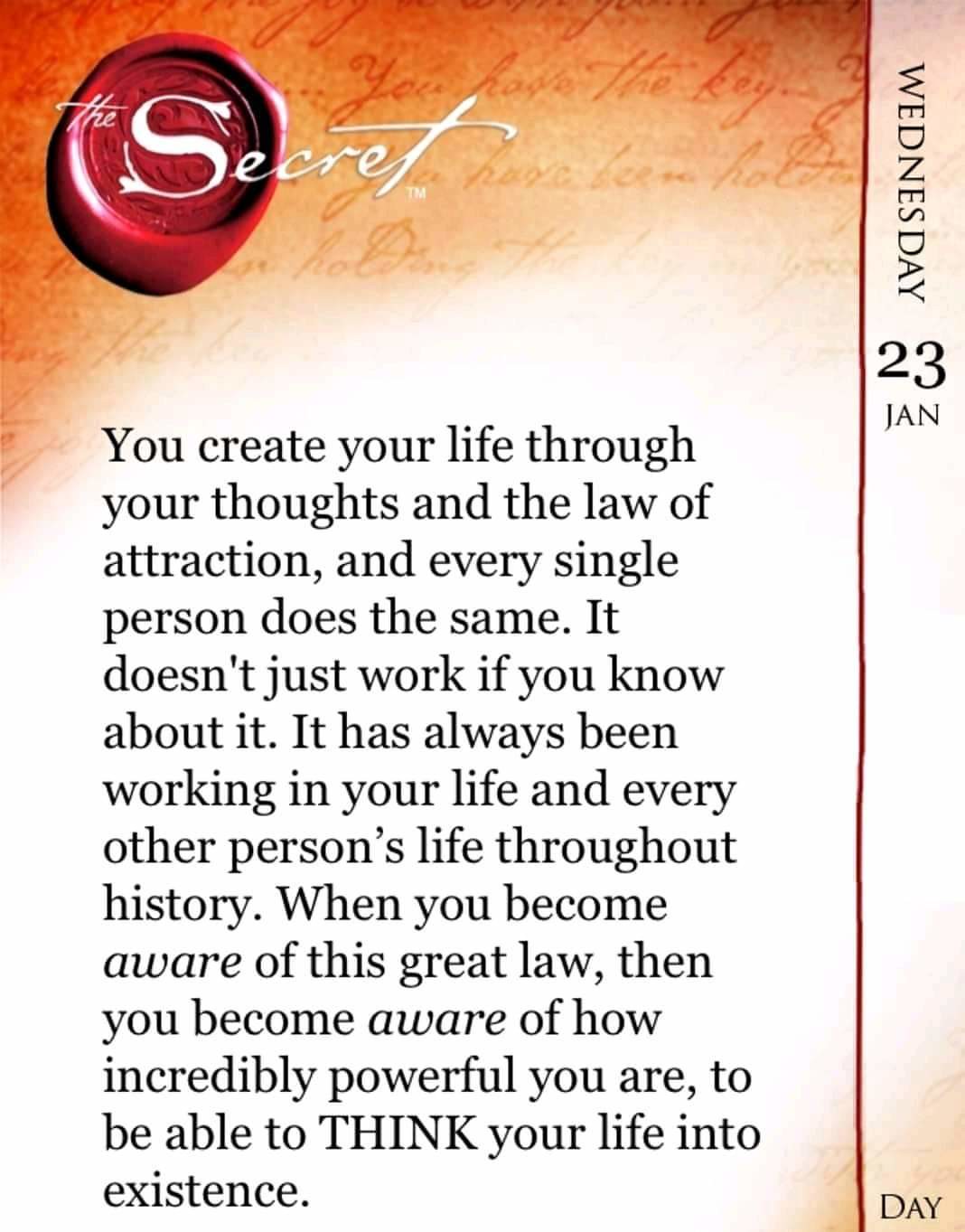The image depicts a passage from a daily calendar or a page from a book, likely "The Secret." The background features a faint, brown script that enhances the text's antique feel. Prominently at the top left lies a red wax seal with an "S" embossed in the center, under a header reading "The Secret." The main text in the center of the image reads: "You create your life through your thoughts and the law of attraction, and every single person does the same. It doesn't just work if you know about it; it has always been working in your life and every other person's life throughout history. When you become aware of this great law, then you become aware of how incredibly powerful you are to be able to think your life into existence." On the right side, a vertical line separates the date details, which denote "Wednesday, 23 January," with "day" written at the bottom right. The colors used are primarily an orangish-red, white, black, light tan, and beige, giving the page an elegant and motivational appearance.